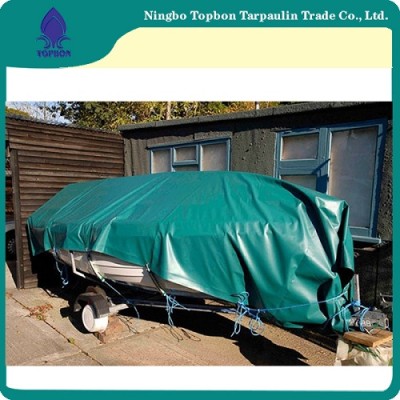The image depicts a backyard scene with a concrete ground and a wooden fence in the background. Adjacent to the fence is a gray shed featuring two blue-framed windows. In front of the shed, a boat is stored on a trailer and covered by a green tarpaulin secured with blue ropes. The hull of the boat, visible beneath the tarp, is white. The backdrop includes tall trees and a sliver of the sky. The entire photograph is framed with green, yellow, and white borders, and a logo marked "TGPBON" is positioned in the top left corner. Additionally, there's a strip of white text on a green background at the very top, reading "Ningbo Tapalin Trade Company Limited." The setting and various elements, including a boat cover, concrete pavement, and shed, suggest an outdoor storage area, possibly within someone's residential property.